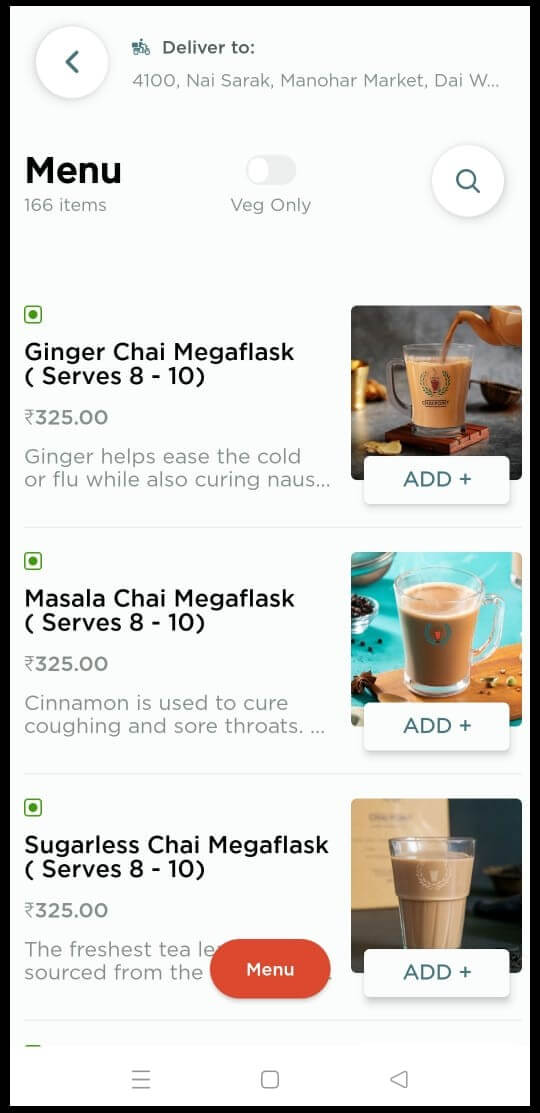In the photograph of the application interface, we see a sleek, modern design set against a clean, white background and outlined in black. The text is also in black, providing a clear contrast for readability. At the top, there is a circular icon featuring a back arrow, indicating the option to navigate back, alongside the delivery address "4100 Nisarak Manohar Market."

Below this, a menu is displayed, listing 166 items available for selection. The "Veg Only" filter has been toggled off. To the right of the menu header, there is a search icon resembling a magnifying glass, allowing users to quickly find specific items. 

A green square icon, containing a smaller circle, is prominently displayed with the text "Ginger Chai Mega Flask" indicating that it serves 8 to 10 people. Adjacent to this, there is a photograph capturing a kettle pouring chai into a glass mug, which is set on a coaster.

Further down, another listing shows "Masala Chai Mega Flask," also serving 8 to 10 people. Accompanying this item is an image of a clear glass mug surrounded by herbs, highlighting the fresh ingredients used.

Lastly, we see "Sugarless Chai Mega Flask," for which a detailed photograph illustrates a glass filled with a rich, brown liquid, representing the chai. Each image and description provides a visual and textual representation of the chai varieties available for order.